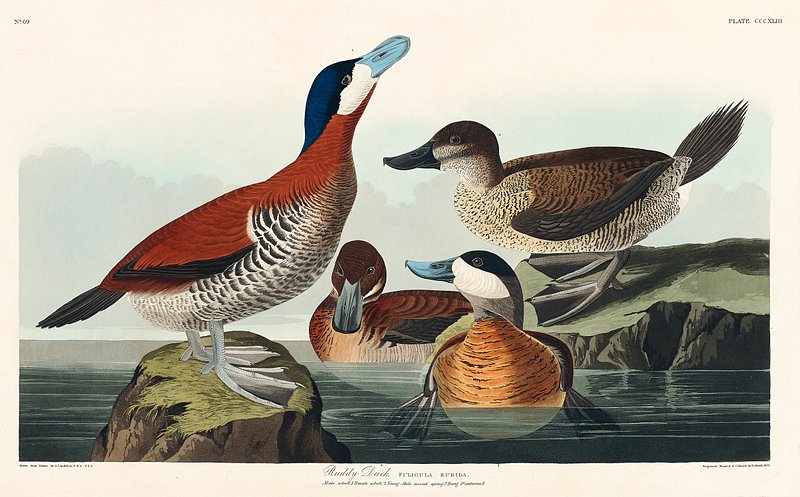This image appears to be an old, possibly valuable print or lithograph featuring a detailed and richly colored depiction of ducks, reminiscent of a Currier and Ives illustration. The scene captures four ducks, each meticulously illustrated with intricate feather details. Two ducks are swimming in the water, where their webbed feet are visible below the surface. The ducks exhibit a vibrant and atypical color palette, including shades of copper, burnt orange, and auburn, with variously colored beaks in blue, brown, gray, and black.

On the left, one duck stands on a small grassy island, displaying a red body with a white and black underbelly and a navy-blue crown, complemented by a robin blue beak. The water in the center contains two ducks; one has an orange belly with a blue beak and the other is an auburn shade with a gray beak. To the right, another duck stands on a rocky ledge, showing brown and cream plumage with a gray underbelly and a black beak.

The background is a muted blend of cream and gray shades with light blue highlights, giving the scene an aged look. At the top left of the image, there are numbers, while the top right has "plate" followed by a Roman numeral. The bottom of the image contains additional text, with fine print on both the left and right corners. This detailed portrayal, combined with the evident age and high-quality coloring, suggests that the print might hold significant value.